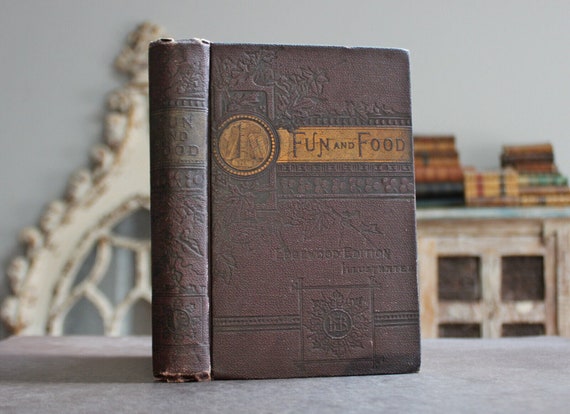In the foreground of the image is a very old, dark brown leather book with intricate embossed designs featuring leaves and flowers. The cover prominently displays a lighter brown rectangle with the title "Fun and Food." Around this title, there is a circle and various indistinct embossed words, including "edition," though the rest of the text blends into the background due to the similar coloring. Below this, a stamp or insignia is present, though it is difficult to discern. The book stands on a gray surface casting a shadow to the left. In the out-of-focus background, there appears to be rustic, worn shelving or an antique cabinet with several old books stacked in three to four piles. Additionally, an interesting, unidentifiable piece of furniture is visible, lending to the overall vintage ambiance of the scene.